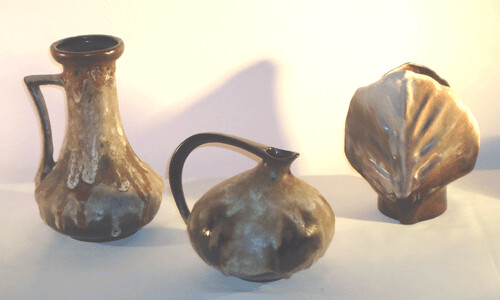This indoor digital photograph features a trio of glazed clay-styled pots, all in various shades of greenish-brown with white speckling, likely owing to age. The background comprises a light-colored wall and floor, with darker shadows cast on the left side due to the light source, and a conspicuous dark spot near the right center.

The pot on the far left is characterized by its tall, slender pitcher-like shape, featuring a wide, open rim that narrows down the neck and flares out at the bottom. It includes a prominent, elongated handle that emerges at a 90-degree angle from the top and reattaches near the base.

The central pot is notably squat and wide, resembling a traditional vessel for holding liquids. It has a narrow spout and a broad bottom, coupled with a U-shaped handle that connects the upper part of the vessel to its midsection.

On the right is a pot shaped intriguingly like a large leaf or shell, with a small base that expands out towards the middle before tapering again at the top. This piece also features an opening at the top.

All three pieces share a consistent glazing technique that combines darker brown tones with mottled lighter browns and whites, enhancing their antique appearance.